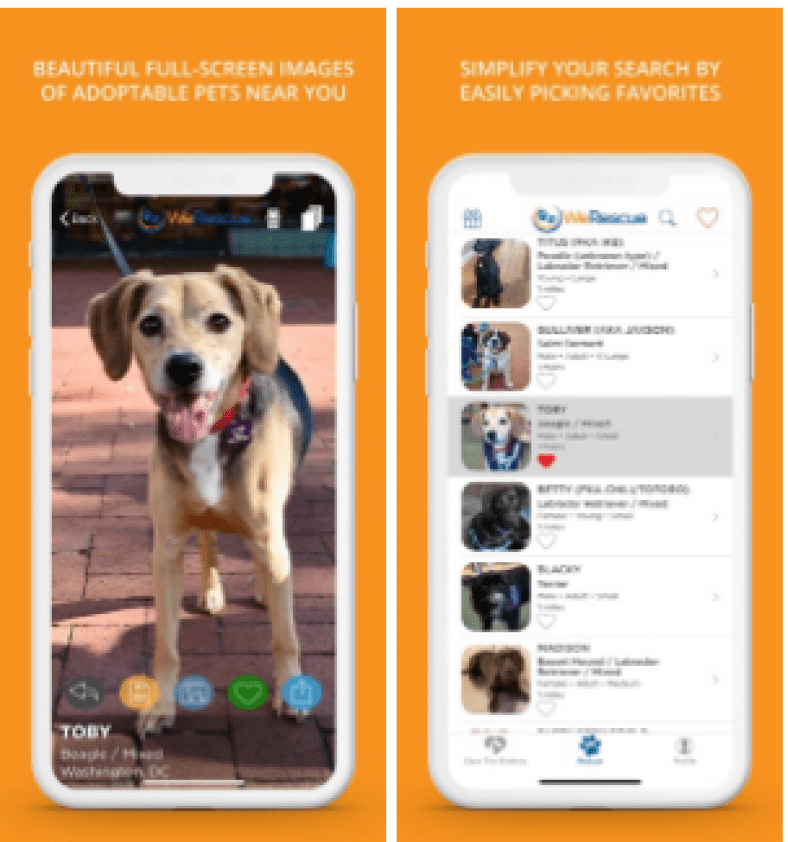Two side-by-side smartphone screenshots showcasing an app designed to help users find adoptable pets nearby. The first screen, set against a vibrant orange background, displays a message at the top: "Beautiful full-screen images of adoptable pets near you." Dominating the screen is an image of an adorable, approximately one-year-old German Shepherd named Toby. A series of icons are positioned at the top, including a backwards arrow, several unreadable icons, a heart, and an upload icon.

The second screenshot, also with an orange background, focuses on simplifying the search for adoptable pets. It shows vertically stacked images of different dogs. The text at the top encourages users to "simplify your search by easily picking favorites." At the top of this vertical list is an image of a black Labrador, followed by a St. Bernard. The third image, highlighted with a heart to indicate it has been favorited, features Toby, the German Shepherd from the first screen. Below Toby, there's a Chocolate Labrador, which is partially visible, and beneath that, the face of a Poodle. The background of this screen is white, and the overall layout of both screens indicates that this app is user-friendly and designed to help find pets for adoption.